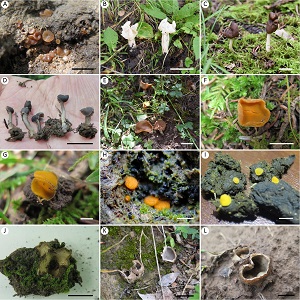This image is a grid composed of 12 separate photos featuring various types of organic materials including mushrooms, fungi, rocks, and plants. The grid is organized in four rows and three columns, with each photo labeled with a letter from A to L in a black uppercase font within a small white circle located in the top left corner of each photo. The first row is labeled A, B, C; the second row D, E, F; the third row G, H, I; and the fourth row J, K, L. The colors in the photos prominently feature greens, oranges, yellows, and mud-browns, with hues like moss green, gray and brownish-yellow tones depicting the fungi. Most of the photos capture natural settings with mushrooms and fungi growing on rocks or amidst moss, except for the photo labeled D, which shows small mushrooms held in the palm of a hand. Overall, the image provides a detailed and colorful representation of various types of fungi and their natural environments.